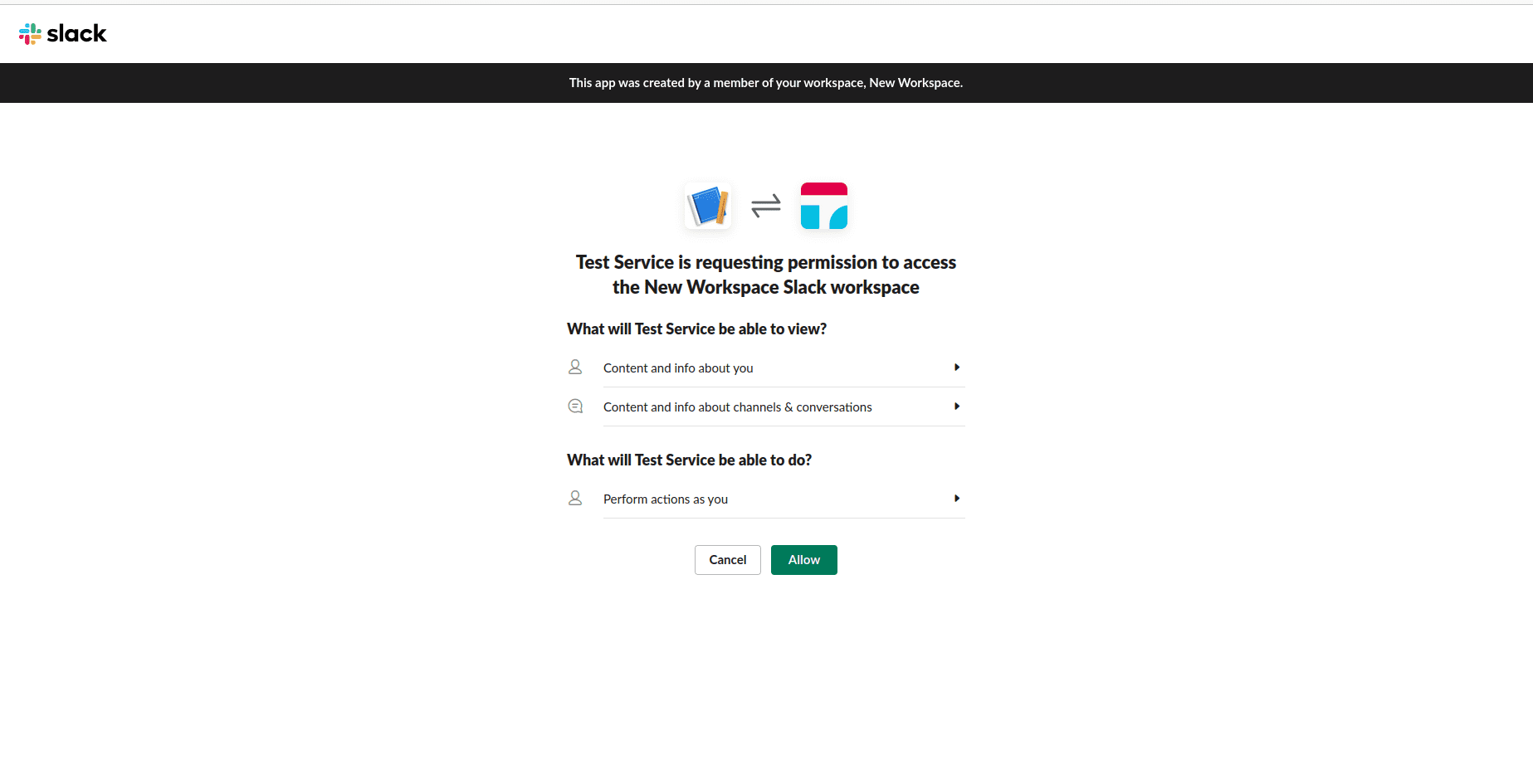This detailed caption describes an image featuring a Slack application permission request interface:

The image showcases a Slack interface set against a clean, white background. Central to the image is a rectangular black bar displaying a picture of an open book and a pencil. Below this, there is a graphic depicting a two-way arrow leading to a white square outlined in blue and red. This visual appears to be part of a permission request from a service named 'Test Service', asking for access to a new Slack workspace.

The content of the permission request is clearly laid out, detailing the specific permissions being requested by 'Test Service'. The service seeks permission to view content and information about the user, as well as content and information about Slack channels and conversations within the workspace. Additionally, the request mentions that 'Test Service' will be able to perform actions on behalf of the user.

At the bottom of the image, there are two clickable options: a white rectangle labeled 'Cancel' and a green rectangle with an action button that appears to start with the letter 'A'. These buttons are intended for the user to either deny or grant the requested permissions.